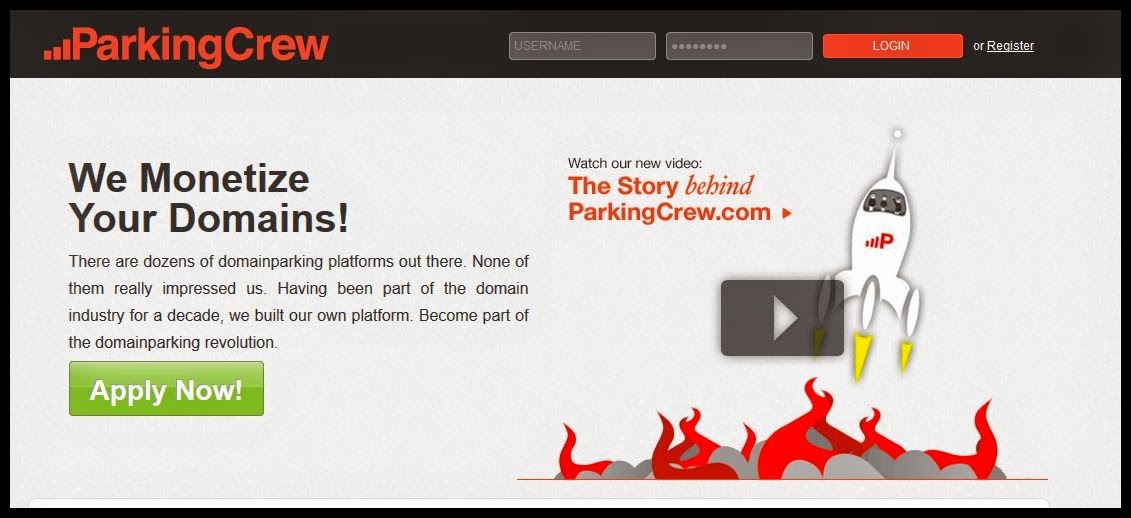The image appears to be an advertisement for a domain parking service. The design features a thicker black banner at the top, extending down the left and right sides as thin borders, and a similarly thin border along the bottom left that reaches across to the right.

Within the top black banner, there's a dark orange section displaying the text "ParkingCrew." To the left of "Parking," the banner features an icon resembling a series of steps or Wi-Fi strength bars. Below this, there is a gray area for users to enter a username and password in separate fields.

Just beneath this, another dark orange section contains white text reading "Log in," and adjacent to it, an underlined "or register."

The main background below these sections is a creamy color. On the left side, a brown text block states, "We monetize your domains. There are dozens of domain parking platforms out there, but none of them really impress us. Having been part of the domain industry for a decade, we built our own platform, becoming part of the domain parking revolution." 

Below this text, a green button with white text invites users to "Apply Now."

On the right side of the poster, there’s a video thumbnail featuring a white spaceship launching from a red planet. The thumbnail text reads, "Watch our new video: the story behind ParkingCrew.com."